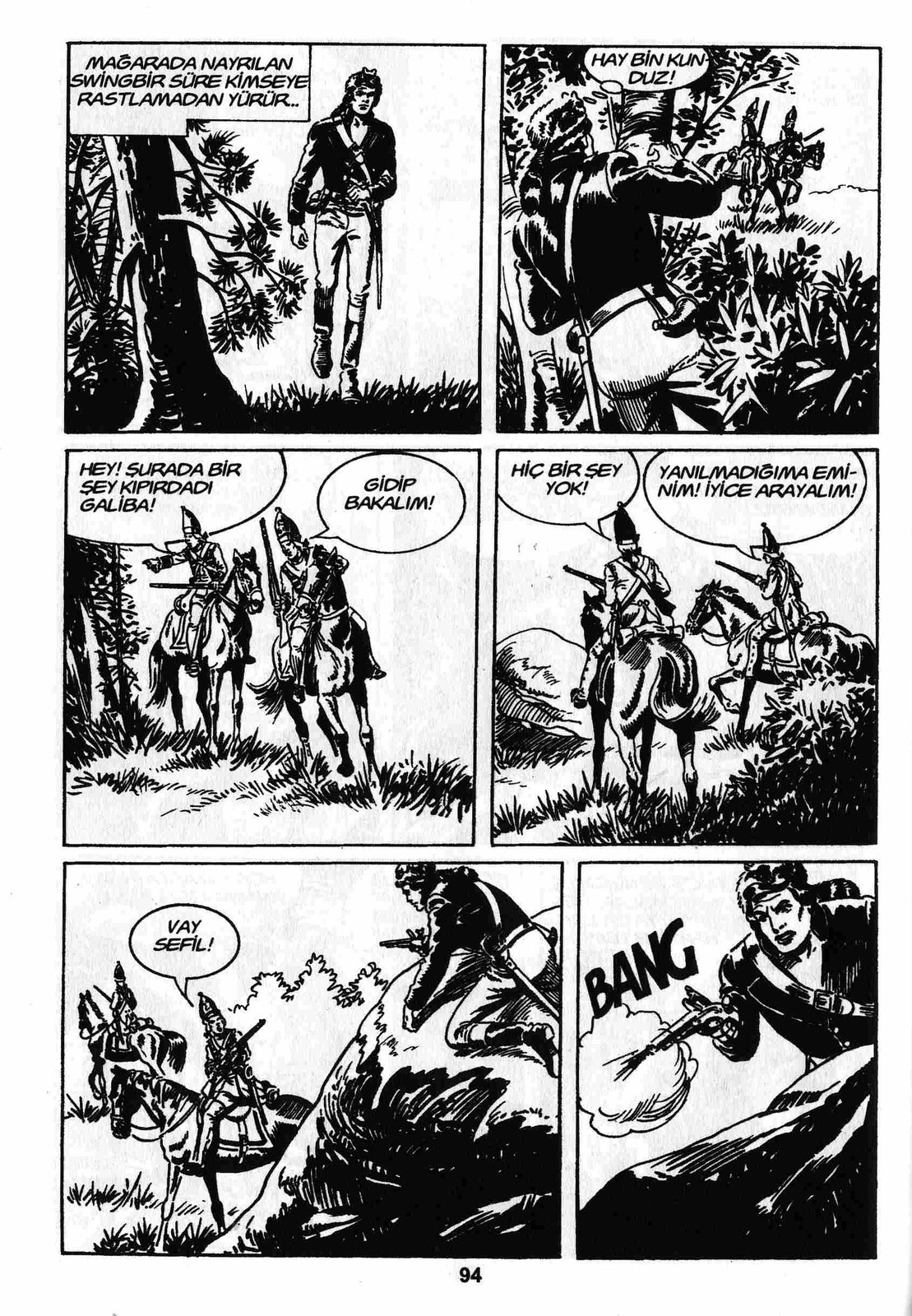This detailed black-and-white comic book page features six rectangular panels arranged in three rows. The comic tells an action-packed story set in what appears to be a Western or frontier setting. The story begins with a long-haired man wearing a coonskin cap, walking through a wooded area in the first panel. He seems alert to his surroundings. In the second panel, he hides behind a tree as soldiers, possibly dragoons in tall hats, approach on horseback. As tension builds, the third panel shows the soldiers spotting him and turning their horses towards him. The fourth panel captures the soldiers, with rifles ready, nearing a set of rocks where the man has taken cover. In the fifth panel, one soldier discovers the man crouching among the rocks, armed with a muzzle-loading pistol. Finally, in the sixth panel, the action culminates with the man firing his pistol, accompanied by a "BANG" in the text. At the bottom of the page, the number "94" is written.